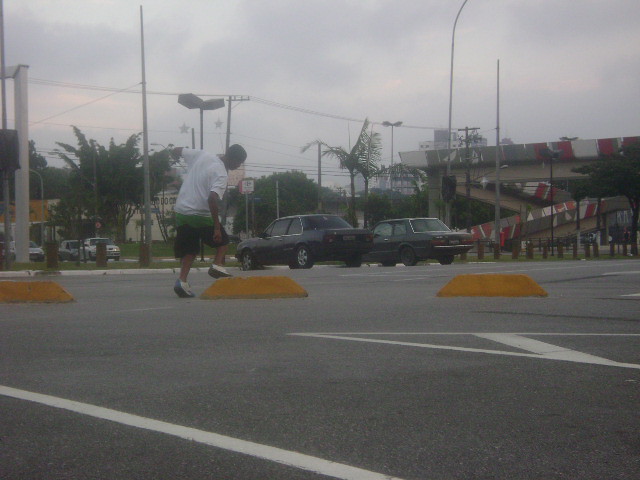The image captures a predominantly empty parking lot beneath a gloomy, gray, and cloudy sky. Central to the picture, a man with dark brown skin is stepping on a yellow parking curb. He is dressed in a white shirt with green accents, black shorts, and white and blue sneakers. Two two-door sedans – one black and one gray – are parked near the center, serving as a focal point. The asphalt ground is marked with white parking lines and additional yellow curbs. In the background, tall palm trees line the sidewalk near the main road, accompanied by power lines, light poles, and a distant traffic light. A parking structure appears in the right corner, and there are visible storefronts, including what seems to be a KFC, and various street signs.